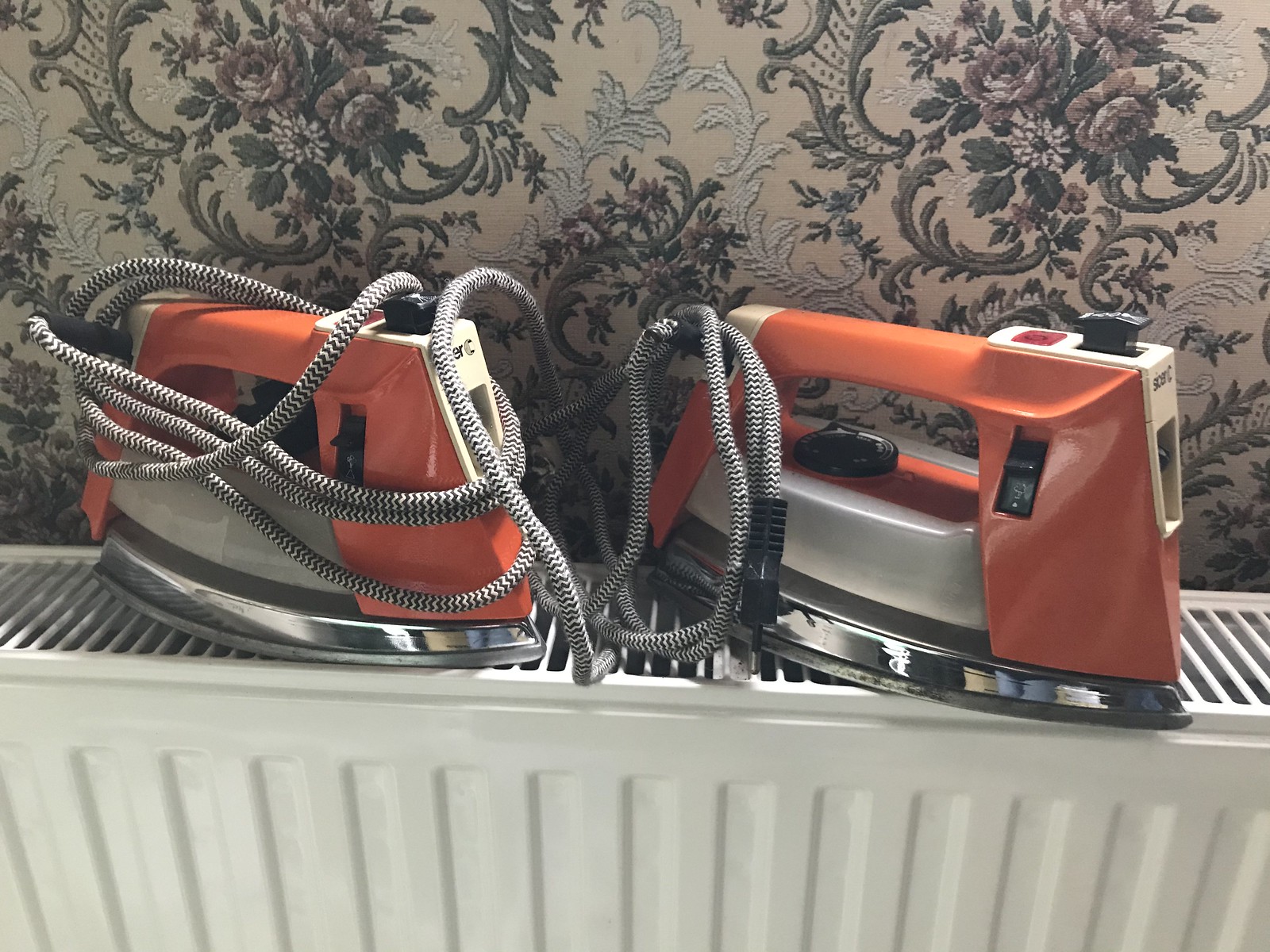The image features two nearly identical retro-style clothes irons positioned side by side on a flat-topped, white radiator. Each iron prominently displays a reddish-orange handle and center with a transparent water tank and a silver chrome base. The cords, appearing coiled and resembling striped black and white or black and gray cloth, are wrapped around the irons. Additional details include large black buttons on the top and side of each iron. The radiator, with visible grating, is set against a cream-colored wall adorned with ornate, flowery wallpaper featuring green and pinkish hues. The overall setting evokes a vintage or old-fashioned ambiance, hinting at a hotel or a traditionally styled home.